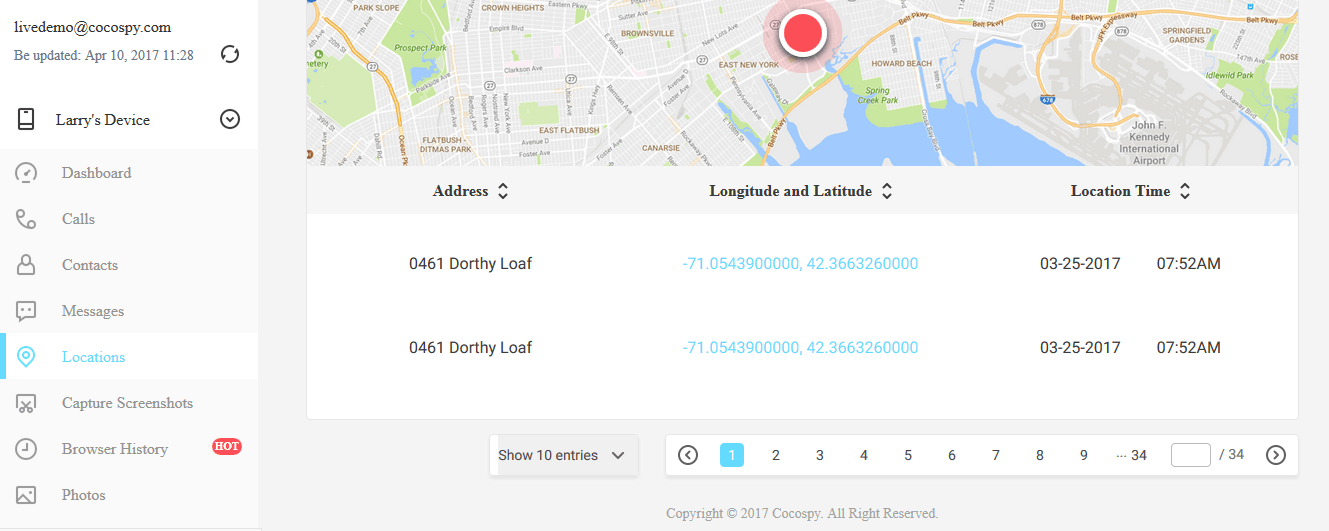Caption: 

"Live Demo at Kokosvp.com: Larry's Revised Smartphone Dashboard

The dashboard comprehensively displays Larry's calls, contacts, messages, locations, captured screenshots, browsing history, and photos. A prominent feature is a large red circle that highlights different street views, water bodies, and various other elements. Key details include specific addresses, longitude and latitude coordinates, and location time points such as: 46.1°N, -71.05° at 07:52 AM on 3rd June, 2017. The entries are numerically organized, with sequential listings from 1 to 34."